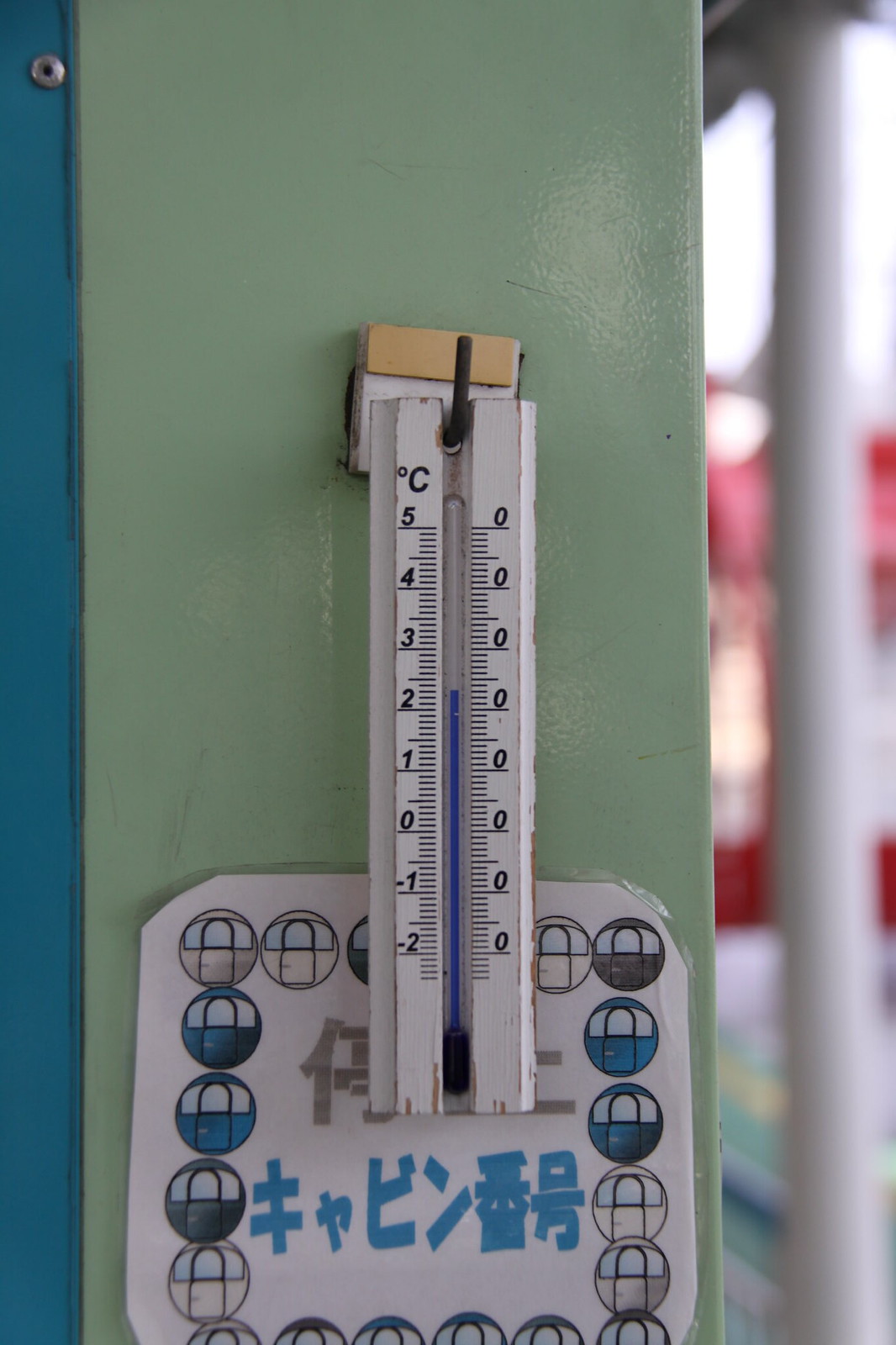This image captures a detailed view of a thermometer mounted on an exterior green wall. Directly beneath the thermometer is a white plaque adorned with light blue and gray text in Chinese characters, as well as a pattern of semi-circles in varying shades of blue, gray, and white. The thermometer itself is white with measurements marked on both sides; on the left side, the scale ranges from -2 to 5 degrees Celsius, with a large "C" at the top indicating Celsius. On the right side, the same numbers are featured, but each is accompanied by black horizontal lines. The setting includes additional elements such as a white post adjacent to the wall and a blurred object in the background that has a reddish-orange hue. The overall color palette of the scene is dominated by greens, whites, and blues.